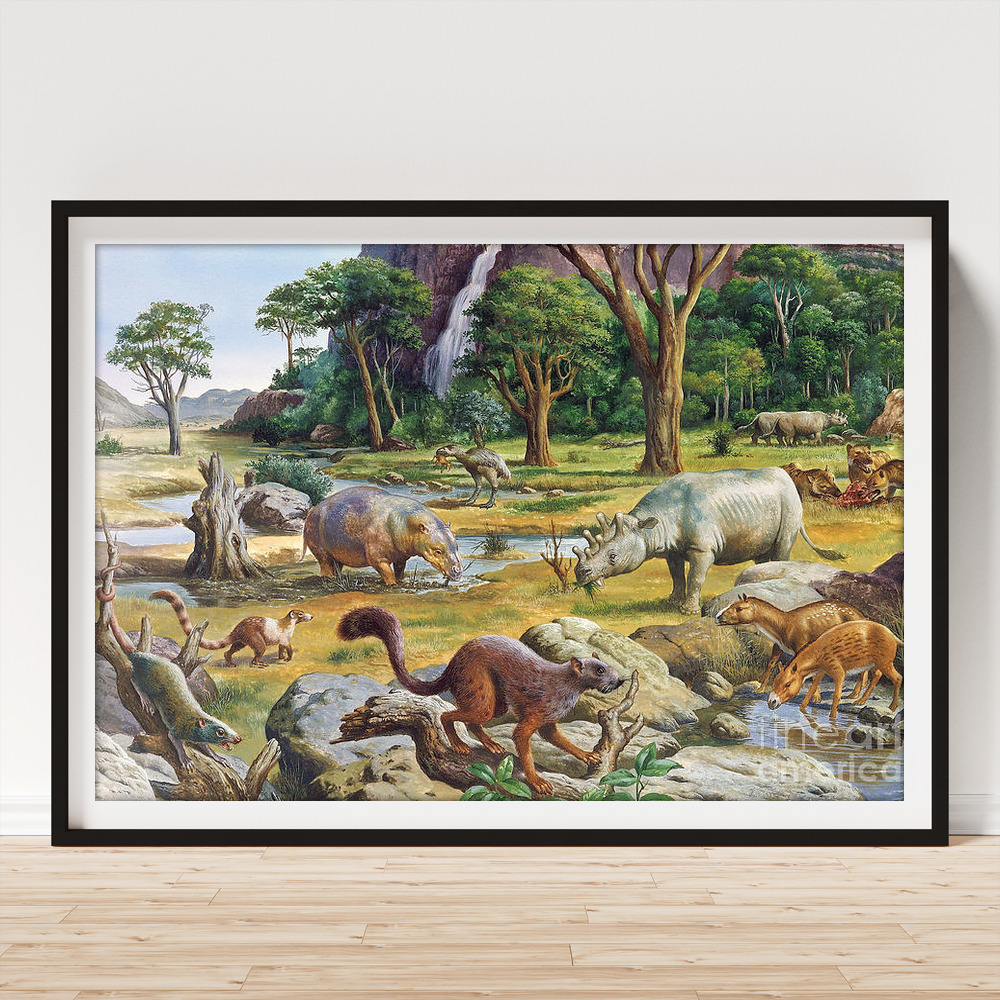The image depicts a framed landscape artwork, mounted on a light-colored table against a white wall. The artwork, titled "Linear America" as noted on the right corner, showcases a vibrant, bustling scene around a watering hole, possibly in Africa. Central to the composition are a hippopotamus and a rhinoceros, standing close together, with the hippo drinking from the water and the rhino grazing nearby. 

Surrounding these large mammals, various smaller animals are visible, including what appear to be rodents or mongoose-like creatures and unidentified long-tailed mammals. Among them, some antelope or deer-like animals drink from a puddle on the right. The middle ground and background reveal a lush environment with numerous trees and a grand waterfall cascading from a steep, tall mountain.

In addition, glimpses of a dinosaur-like bird holding a small animal in its beak and lions feasting on a carcass add a mythical touch. The scene is dotted with animals that seem both familiar and exotic, some even reminiscent of extinct species, contributing to the artwork's enchanting and timeless quality. The overall vibrant gathering of diverse fauna against a richly detailed natural backdrop creates a visually captivating and dynamic composition.